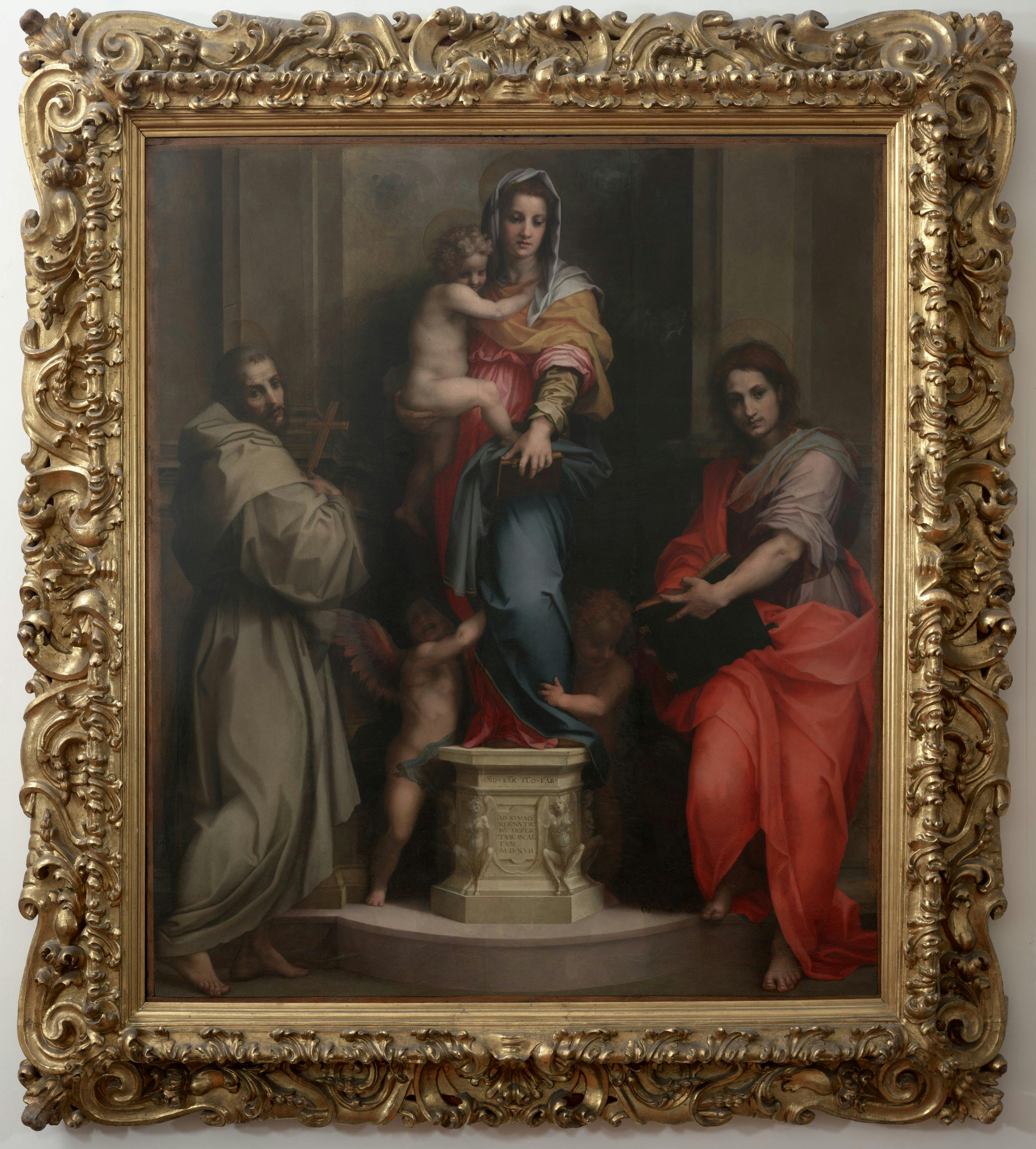The painting is displayed on a very light gray wall, casting subtle shadows from its highly ornate, aged golden frame adorned with intricate carvings and swirls. The central figure in the image is a woman, seemingly from biblical times, standing on a pedestal and dressed in layered rags while cradling an undressed baby. At her feet are two children, also unclothed, who cling to her legs. To her left, a person dressed in a red robe over a tan shirt holds what appears to be a Bible or scroll. On the right, a man in a tan, flouncy robe stands with a brown cross cradled in his arm. Both the man and the woman have their arms outstretched, adding to the composition's dynamic feel. The scene evokes a classical religious tableau, potentially depicting Christ, Mother Mary, and cherubic figures in a spiritually significant gathering.